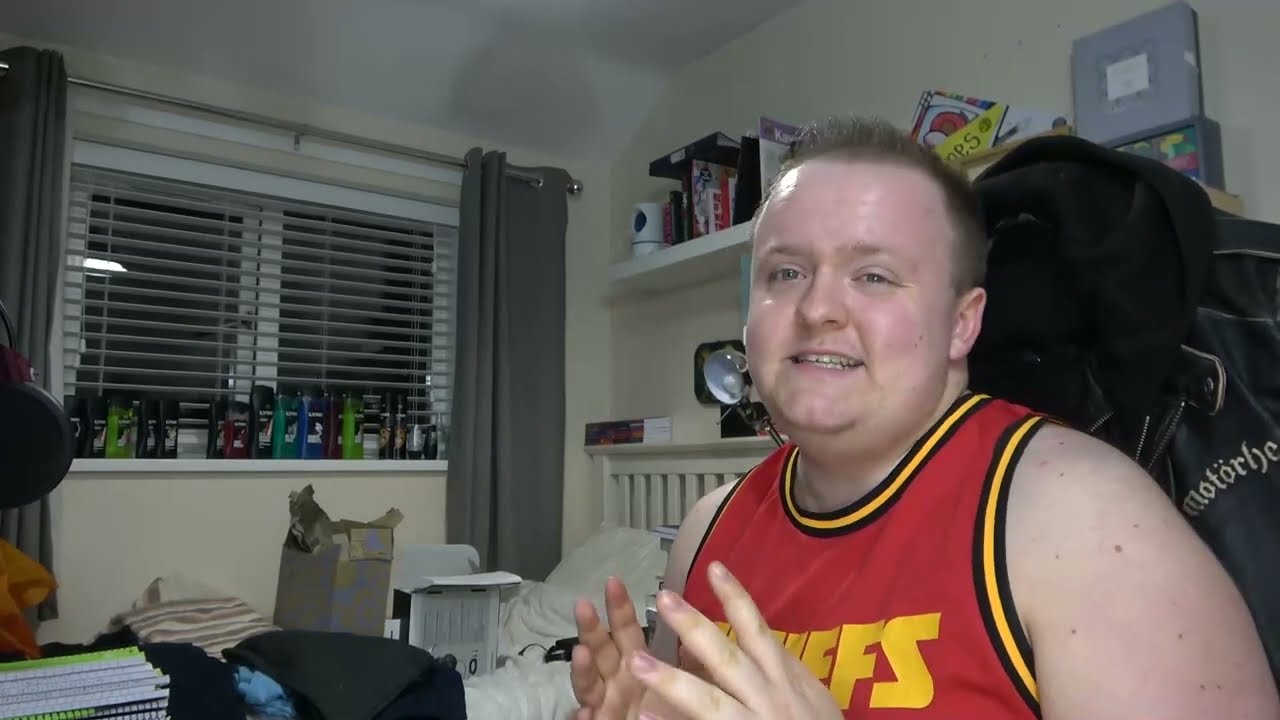The image depicts a somewhat overweight, white male with short blonde hair and no facial hair, sitting in a chair positioned to the right-hand side of the photo. He is wearing a red basketball jersey with the word "Chiefs" emblazoned on it. Draped over the back of his chair is a black leather jacket featuring the Motorhead logo. The man is looking directly at the camera with a smile, and his hands are raised, suggesting he is in mid-conversation or perhaps recording a podcast. 

The setting is within a cluttered bedroom. Behind him, there is a bed piled with boxes, papers, and journals, along with a shelf above it crammed with books. The room features cream-colored walls and a white ceiling. A large window, with shades open, forms the backdrop. The window sill is lined with an assortment of body wash bottles and several packs of deodorant and Axe body spray. The scene, devoid of any readable text, exudes a sense of casual, lived-in disarray, likely captured in the middle of the night.